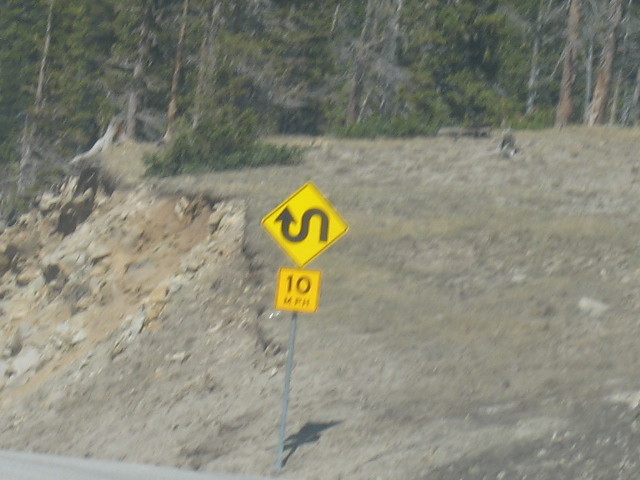The blurry color photograph appears to be taken from a moving car, capturing a rugged landscape. At the top, tall timbers, a mix of hardwood and conifer trees, stand against what seems like the dry terrain, possibly indicative of the western or northwestern United States. The scene shows a hillside descending towards the road, dotted with rocks and short, brown, dying grasses. To the left, the hillside is severely eroded, with dirt and rocks sliding downward, almost reaching the road's edge, a small sliver of which is visible in the bottom left corner.

The day is exceptionally sunny, with bright light flooding the photo. Shadows cast by objects are minimal and directly underneath, suggesting the sun is high overhead. In the center of the photograph, a yellow caution sign commands attention. The sign features an extraordinarily curvy arrow that starts on the right, loops up and down resembling a lowercase "n," finally forming an S-curve with an arrow at the top. Beneath this, a smaller yellow square sign indicates a speed limit of 10 mph, warning of the treacherous, winding road ahead.